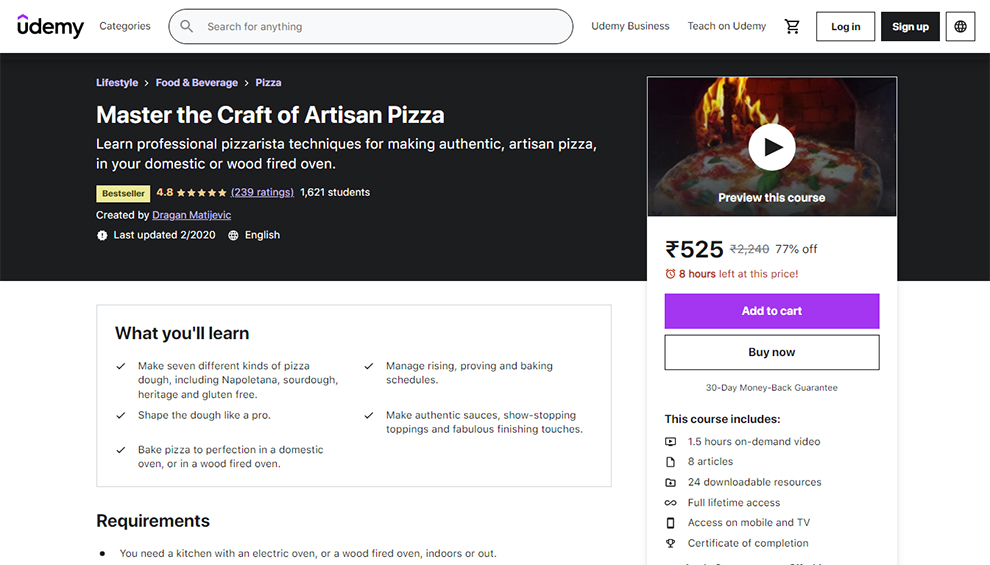**Detailed Caption for the Udemy Course Image:**

The image features the user interface of the Udemy website in a horizontal layout. Starting from the upper left corner, the word "udemy" is displayed in all lowercase with a purple float accentuation over the "u". To its right, the word "categories" is placed next to a search box. Further on the right, there are options for "Udemy Business" and "Teach on Udemy", followed by buttons for "Login" and "Sign Up".

Occupying the central portion of the image is a large horizontal black banner. At the top of this section, small purple text reads, "Lifestyle > Food & Beverage > Pizza". Beneath this, in prominent white bold font, the course title "Master the Craft of Artisan Pizza" is displayed, followed by the subtitle detailing the course content: "Learn professional pizzerista techniques for making authentic artisan pizza for your domestic or wood-fired oven."

Below the subtitle, a yellow horizontal rectangle labeled "Bestseller" is prominently featured in dark text. Adjacent to this banner in orange text, the course rating is shown as "4.8" accompanied by nearly fully colored five stars. In purple, the number of ratings "(239)" is noted alongside the number of enrolled students "1,621" in white.

Continuing down, the text "Created by" precedes the author's name, and additional white text indicates the most recent update of the course. Below this, in black font, the section "What you'll learn" is listed in a horizontal rectangle outlined in light gray. The learning outcomes are divided into two columns, with check marks preceding each item:

- First column:
  1. Make seven different kinds of pizza dough, including Napolitana, sourdough, heritage, and gluten-free.
  2. Shape the dough like a pro.
  3. Bake pizza to perfection in a domestic oven or in a wood-fired oven.
- Second column:
  1. Manage rising, proving, and baking schedules.
  2. Make authentic sauces, show-stopping toppings, and fabulous finishing touches.

Subsequently, bold black text "Requirements" is followed by a bullet point stating in non-bold black font: "You need a kitchen with an electric oven or a wood-fired oven, indoors or out."

On the right side of the image, partially overlapping the black horizontal banner and the white section below, is a vertical promotional box. At the top is a thumbnail image with a white play button (white circle with a triangle pointing to the right) and the text "Preview this course" in white underneath. Below the preview, a price indication shows the foreign currency 525 crossed out with a 77% discount, reducing the price. In red text, there is a note "8 hours left at this price". At the bottom of this box are two buttons: a purple "Add to cart" button with white text and a "Buy now" button.

Finally, the bottom of the right vertical box lists what the course includes, each preceded by an icon:
- 1.5 hours on-demand video
- 8 articles
- 24 downloadable resources
- Full lifetime access
- Access on mobile and TV
- Certificate of completion